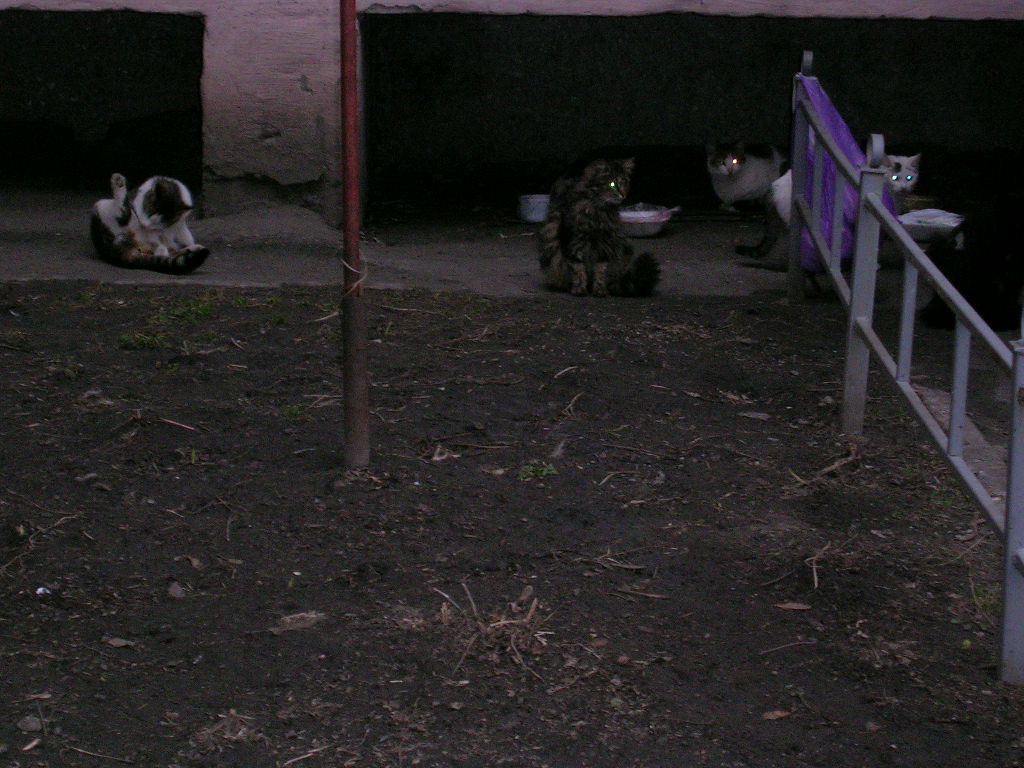In this nighttime photo, a rectangular area is divided into a dirt foreground and a concrete background. On the left-hand side, a long metal gate extends towards the back, ending with a purple trash bag partially obscuring one cat. A vertical pole stands just right of center, its base gray and top red, weathered with rust. 

The dirt area in the front transitions to concrete in the background, where four cats are positioned. The first cat to the left of the pole is a calico with brown and tan fur, yellow eyes reflecting the camera flash, and a thick, furry tail curved behind it. Two white bowls for cat food can be seen nearby. To the right of the calico, and partially obscured by the purple bag, another cat shows just its head, back, and tail; its eyes are greenish-yellow, and it has a black spot on its head, a mostly white face, and a black tail.

A black-and-white cat is to the right of a concrete column in the back, with its head black, a white chest and neck, and raised, splayed back legs as it licks its tummy. The final cat in the far back is predominantly white with black markings around its eyes and on its back. It's a rounder cat, also with eyes reflecting greenish-yellow in the dark.

The setting is minimally lit, resulting in the cats' eyes reflecting sharply in the camera's flash, adding a haunting yet intriguing quality to the scene.